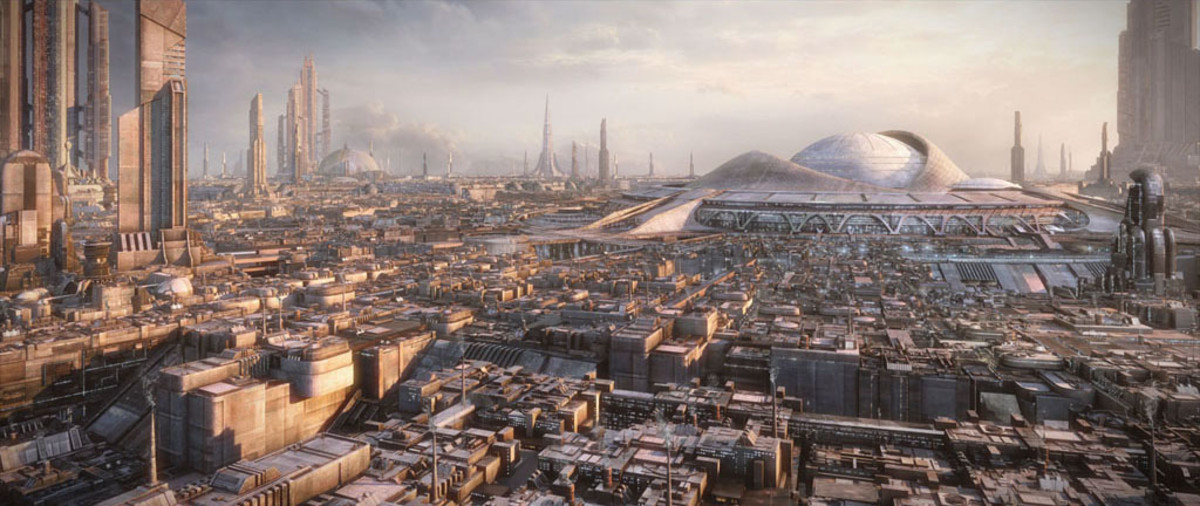This image is an artist's interpretation of a futuristic cityscape, dominated by shades of brown, white, and gray. The sky above is a mix of gray and blue tones, heavily veiled with smog and wispy clouds. The skyline is densely packed with numerous tall skyscrapers, particularly on the left and right edges of the image, which appear brown and lack greenery. 

A prominent feature is a unique domed building situated towards the upper right center of the image. This structure, which evokes a sense of a globe or an observatory, has a large white dome that extends upwards, resembling a massive egg. Another dome, with an open-roof design, appears in the upper left center, surrounded by tall brown skyscrapers.

The foreground is filled with an array of densely clustered buildings in shades of gray and brown, and no roads are visible. Along the horizon, numerous factories emit smoke, adding to the overall sense of industrial activity and contributing to the smoggy atmosphere. The entire cityscape presents a stark, densely packed urban environment devoid of greenery, emphasizing an industrial and futuristic aesthetic.